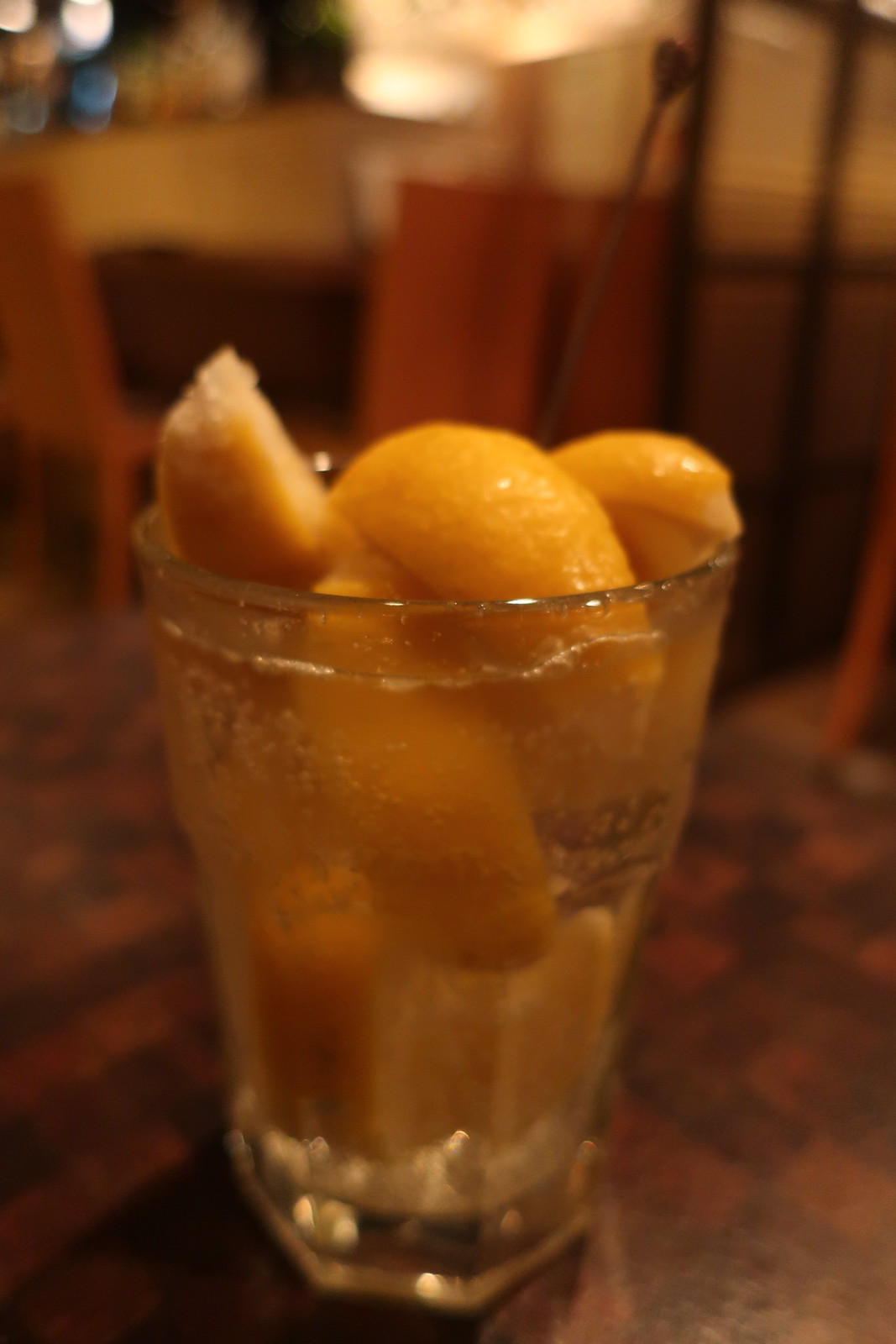In a bustling restaurant setting with a background that fades into a soft blur, a crystal clear glass takes center stage, sitting atop a dark brown, possibly parquet wood table. Inside the glass, a sparkling soda or club soda fizzes, filling the space almost to the rim. The drink is remarkable, not only for its effervescence but also for the abundance of lemon wedges—six in total—that cram the glass from bottom to top, with a few protruding above the rim. Each lemon wedge, a vibrant yellow, is distinctly visible within the drink's clarity, and a brown skewer is tucked inside, potentially for stirring. The glass and its contents are sharply in focus, contrasting with the indistinct blur of tables, chairs, and ambient lights in the background, adding an air of mystery to the setting.